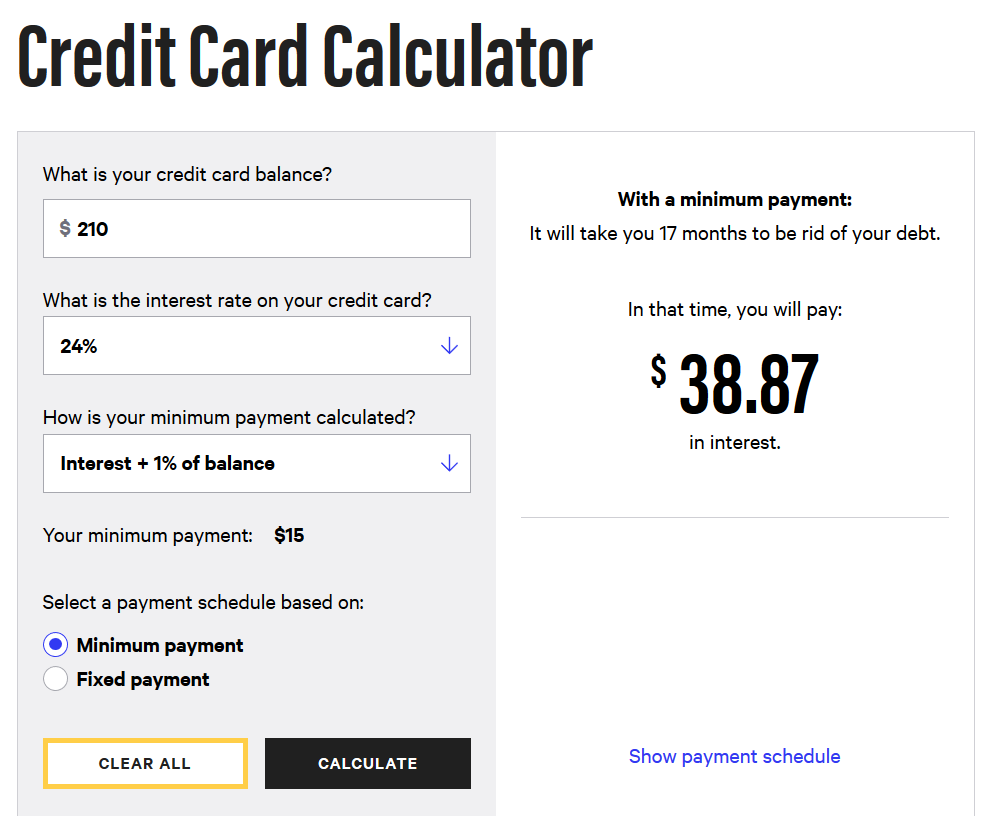This screenshot displays a credit card calculator interface. The title "Credit Card Calculator" is prominently shown in large font on the upper left-hand side, with each word starting with a capital "C." The interface is divided into two main sections: an input block on the left and a results block on the right.

In the left input block, users are prompted to fill in three fields. The first field asks, "What is your credit card balance?" with the user having entered "$210." The second field inquires about the interest rate on the credit card, with "24%" entered as the response. The third and final field asks, "How is your minimum payment calculated?" to which the user has input "Interest plus 1% of balance."

The right results block displays the outcome of the entered information. It states that under the provided conditions, the user will incur "$38.87" in interest over the specified period.